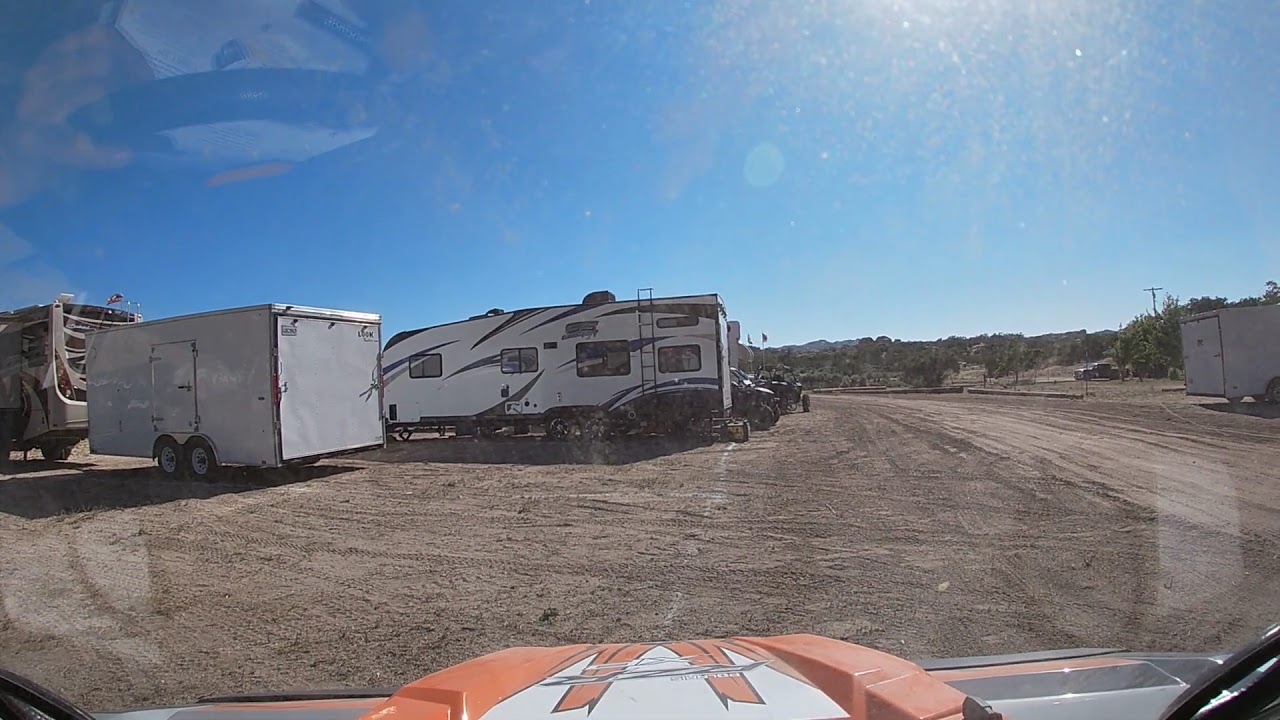The image depicts a vast dirt lot populated with numerous white trailers, suggesting it might be a campsite, trailer park, or rest station for parked trailers and campers. Central to the scene is a larger trailer, behind which several off-road ATV vehicles, predominantly black in color, are noticeable, though somewhat indistinct. To the right, a black pickup truck is visible in the background. The terrain is primarily a dirt field bordered by green shrubs, with a few patches of grass visible further back. The sky is exceptionally clear and blue, adding to the bright, naturally lit setting. The photo seems to be taken from inside an orange, white, and black off-road ATV vehicle, possibly by the photographer. The overall atmosphere portrays a serene, open space with minimal distant features.